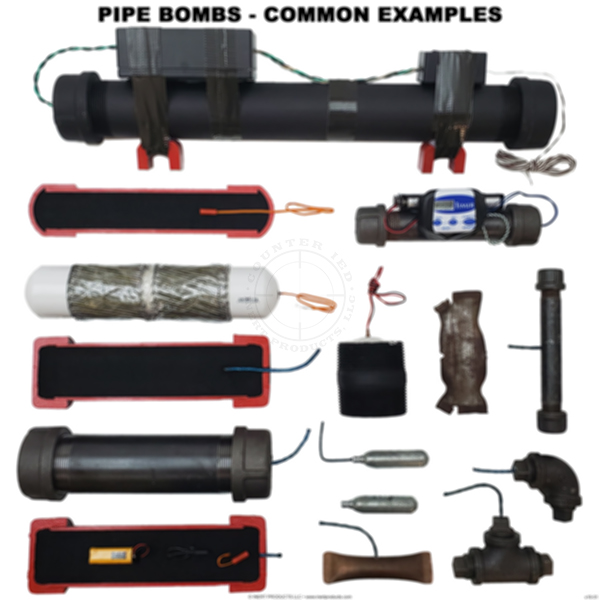The image titled "PIPE BOMBS - COMMON EXAMPLES" in bold black print showcases a variety of different pipe bombs, demonstrating various designs and configurations. At the top of the image, there is a long tubular pipe bomb on red feet with a wire extending from it, setting a prominent example. Below it, to the left, five medium-sized circular tubes equipped with wires are neatly aligned. To the right, a medium-sized pipe bomb, potentially with a small camera, sits above another round device with a fuse resembling a grenade. Adjacent to it, there's a slender pipe bomb, whereas further down, two tiny hot dog-shaped pipe bombs and another medium-sized one can be observed. These bombs exhibit a range of black with red, blue, white, and orange details, highlighting diverse wire configurations and battery placements, often with wires extending either from the top or the side. The assemblage of these pipe bombs is spread across the page, creating an illustrative guide to common examples of such devices.